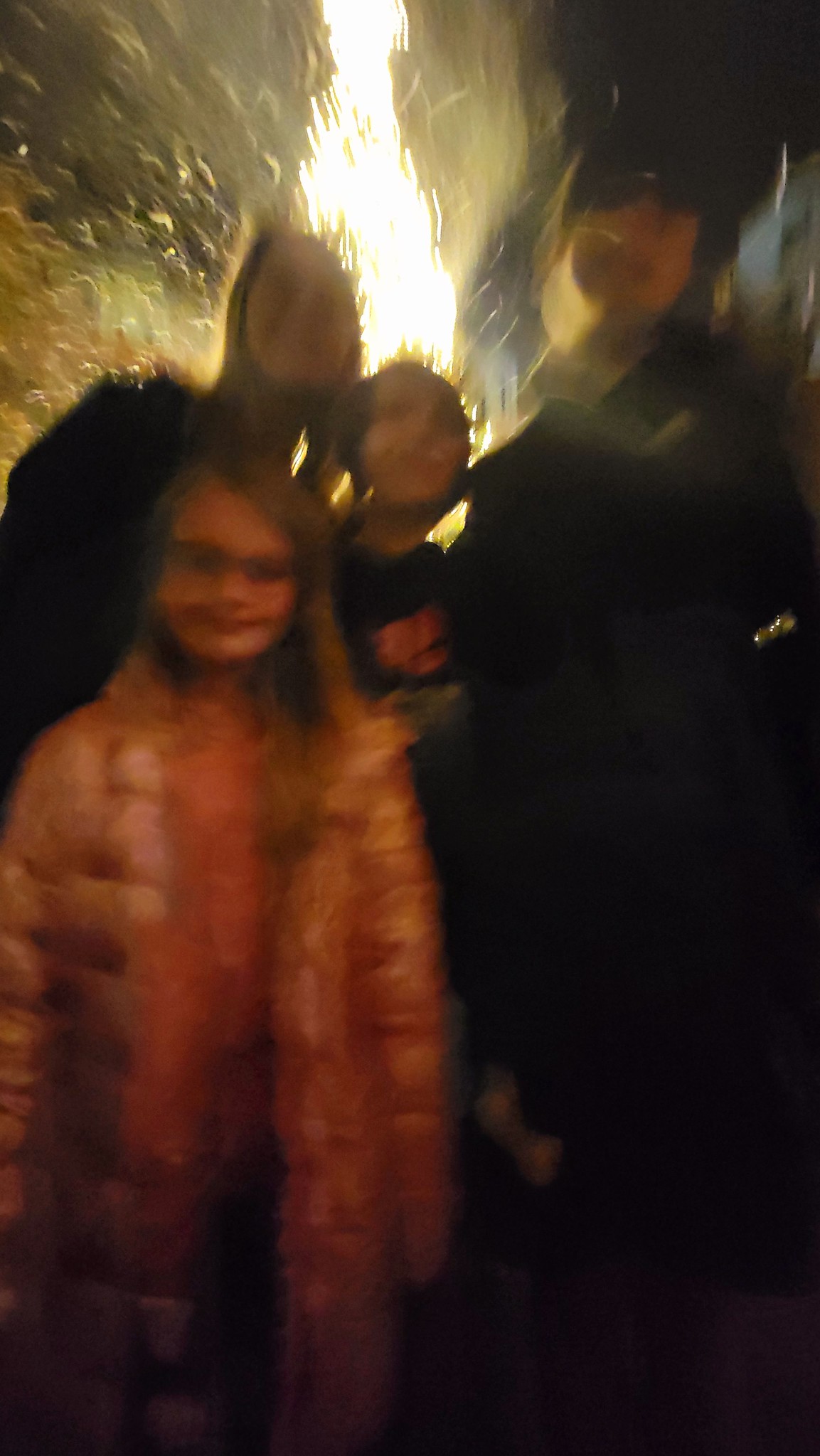A blurry nighttime photo captures a group of four people standing in front of a roaring bonfire. In the foreground is a little girl with long blonde hair, wearing glasses and an open pink puffy jacket. Behind her, a woman, a smaller child, and a man, all dressed in black, stand close together. The man, positioned on the right, wears a black hat and sports a mustache. The woman, standing on the left, leans slightly towards the child in the middle, who is wearing a black shirt adorned with a red emblem. In the background, bright flames shoot up, illuminating the night sky.